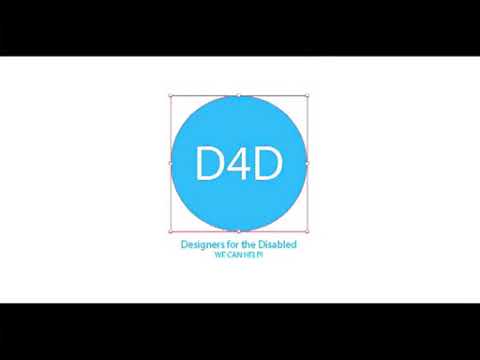This image appears to be a social media screenshot, possibly from Facebook or YouTube, featuring a prominent logo. The focal point is a centered blue circle with the white text "D4D" in the middle. Surrounding the circle is a thin, black square, giving it the appearance of a selected object in design software, such as Photoshop. The background is solid white, bordered by two thick black bars at the top and bottom. Directly below the circle, there is green text that reads, "Designers for the Disabled," followed by smaller, somewhat blurry and illegible text that likely reads "we can help." The overall image suggests an organization dedicated to providing design services for those with disabilities.